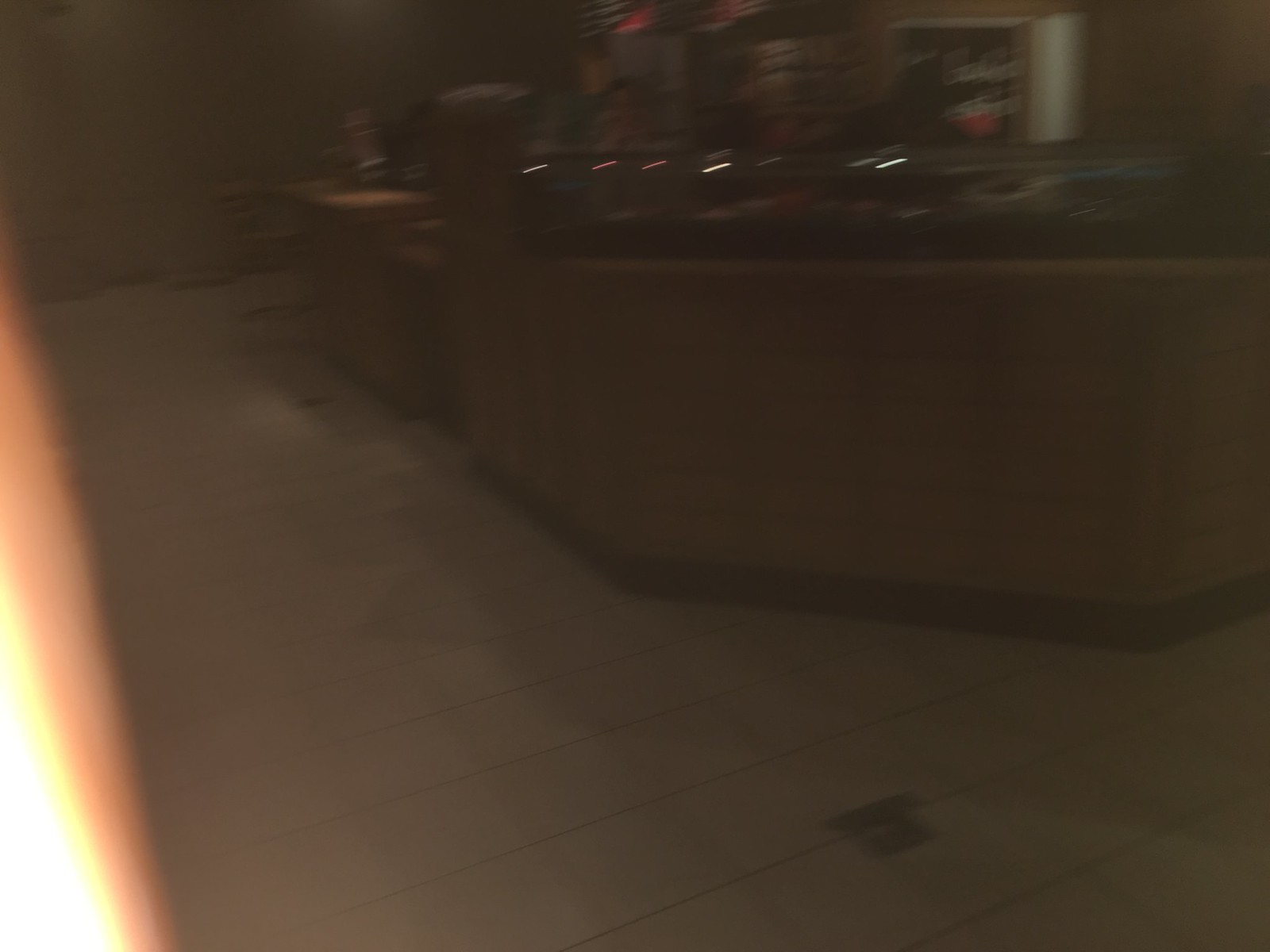The image depicts a cozy restaurant interior within a building. The floor is covered in light-colored tiles. Dominating the foreground is an inviting wooden counter, adorned with intricate small designs that add character to its rich brown surface. A sleek black floorboard trim outlines the base of this wooden structure. Surrounding the counter is a high chair, suggesting a bar-like area for patrons to sit and enjoy their meals. Above the counter, there is a glass display case, likely showcasing a variety of food items available for selection. The overall ambiance hints at a welcoming and thoughtfully designed dining space.